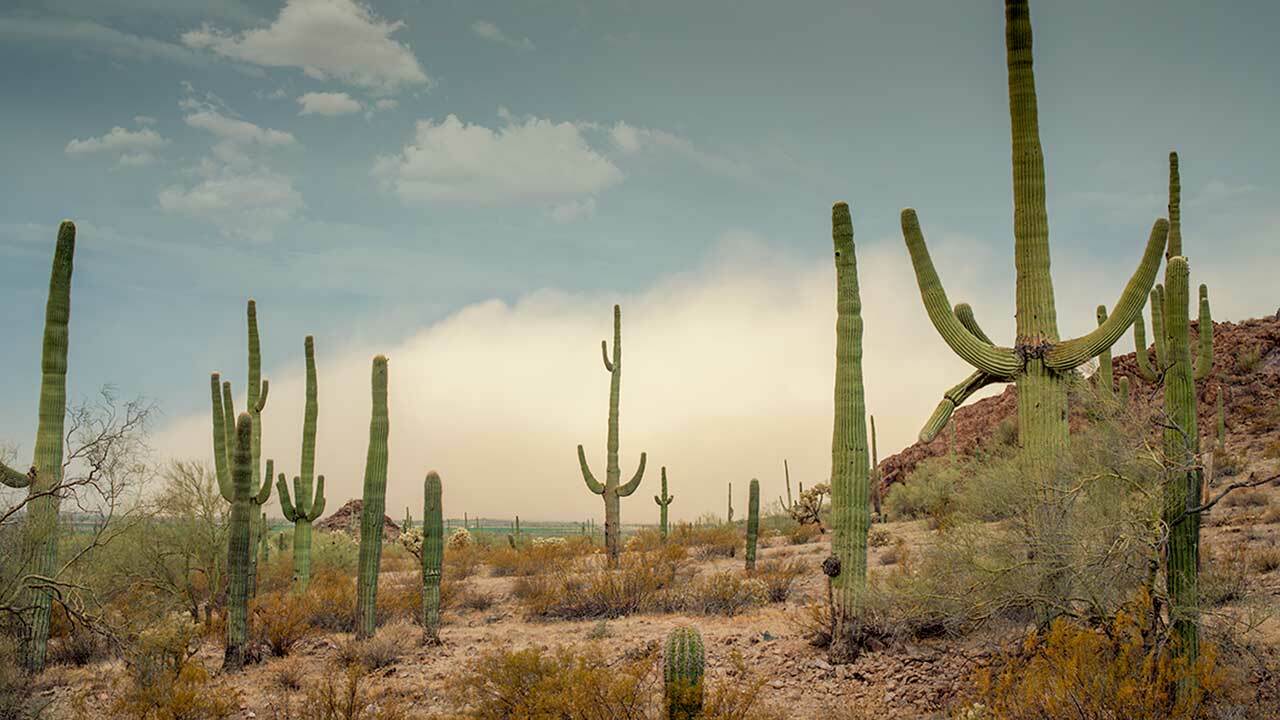This photograph captures a quintessential desert landscape scene, prominently featuring a variety of cacti scattered across the bottom third of the frame. The rocky, beige ground is peppered with sparse patches of reddish-brown grass and scrubby bushes. In the distance, a red rock hill arches from the center to the right, tapering upward against a pale blue sky. This sky hosts a large, arching white cloud near the horizon, accompanied by several smaller, puffy clouds to the left. A subtle green horizon line is visible beneath the large cloud, marked by a small brown hill and some distant green trees. The cacti, primarily barrel cacti with vertical stripes and large arching arms, stand out with their pale green color, some just sprouting close to the ground. The overall scene exemplifies a sunny, serene desert landscape with no animals in sight.